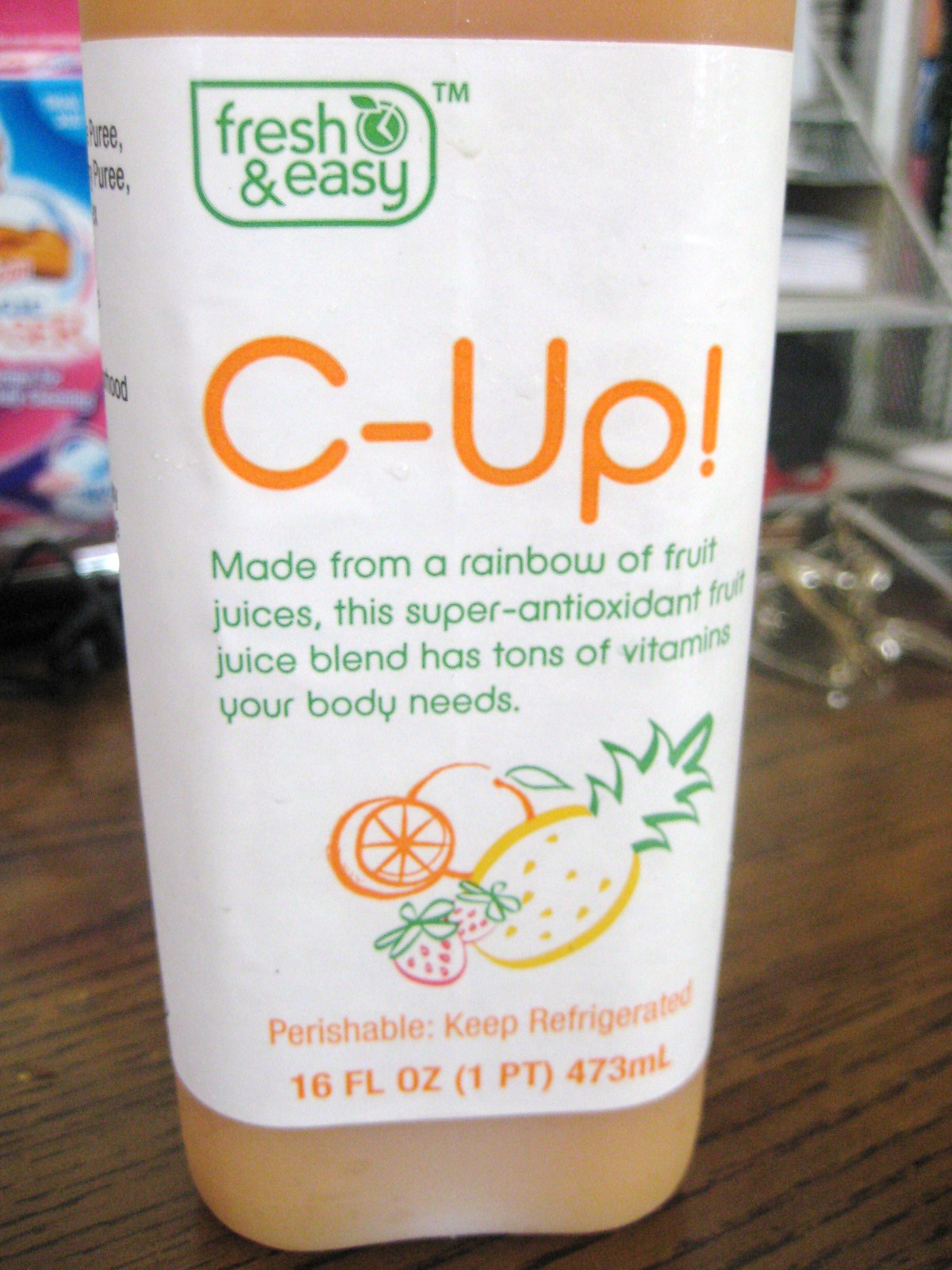A Fresh and Easy product, this “See Up” super antioxidant fruit juice blend is crafted from a variety of fruit juices. The vibrant packaging prominently features artistic sketches of an orange, peach, strawberries, and pineapple, conveying its fruity essence. This 16-fluid-ounce beverage, housed in a translucent plastic container, boasts a multitude of vitamins essential for your body’s needs. "Keep refrigerated" is clearly indicated, emphasizing the perishable nature of the juice. The container rests on a wooden table, surrounded by various items. To the left, a blue, red, and white snack bag with an indistinguishable picture sits partially obscured, and nearby, a set of car keys can be seen. The backdrop reveals a desk and shelves, adding context to this organized and multi-functional space.